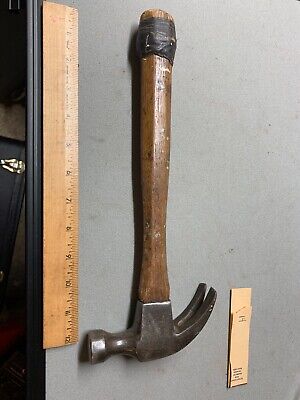In the image, we see a top-down view of a hammer resting on a light gray surface. The hammer is positioned with its handle at the top and its head at the bottom, making it appear upside down. The handle is made of dark brown wood and has a cylindrical shape. At the very top of the handle, there is a black rubber ring—or tape—wrapped around it. The handle extends downward to meet the hammer's head, which is composed of a dark gray, silvery metal. The head of the hammer has a cube-like form with a knob protruding from the left side and two metallic claws extending from the right.

To the left of the hammer lies a brown wooden ruler, positioned vertically with its measurement markings facing the hammer. Adjacent to the ruler, on the far left, there is a black plastic object running from the top to the bottom of the image. Near the claw part of the hammer on the right side, there is a small beige piece of paper. All these objects are arranged against the light gray background, providing a clear contrast that highlights their details.